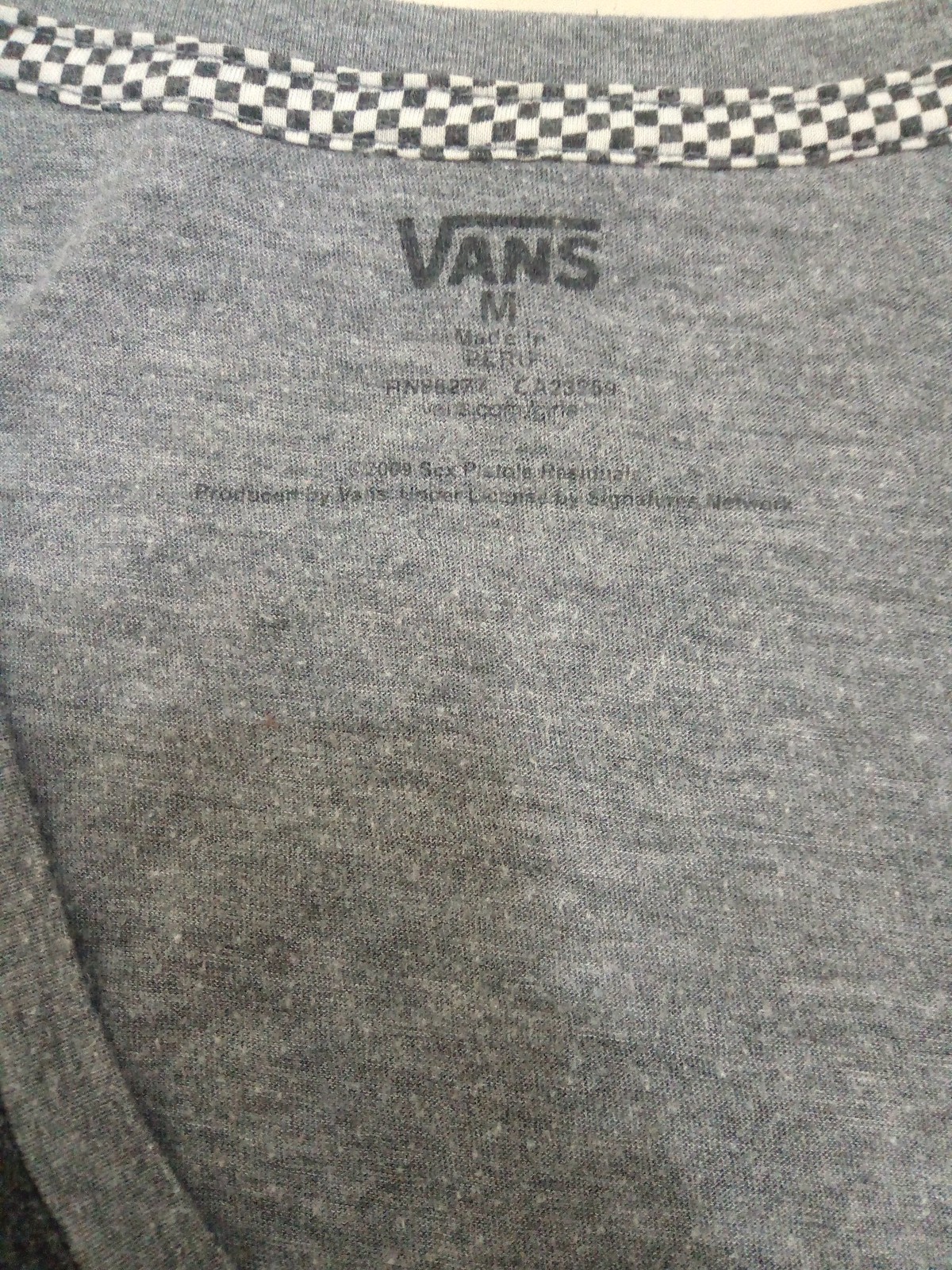This image depicts the inside of a gray Vans t-shirt turned inside out. Prominently featured at the collar is a distinctive black and white checkerboard strip of fabric, stitched on horizontally, which is characteristic of the Vans brand. Centered below the collar, the text "Vans" is printed in black with the iconic long line over the "v" extending above the "a" and "s." Below "Vans," the shirt displays the word "Medium," also printed in black. Further down, there is a faded inscription reading "Made in Peru" followed by "RN86277" and potentially "CA23259." Additional unreadable text and a mention of "2009 Sex Pistols" and "Produced by Network" can be partially made out. The shirt also has a sizable black stain located near the left side, stretching towards the center, resembling an oil stain.